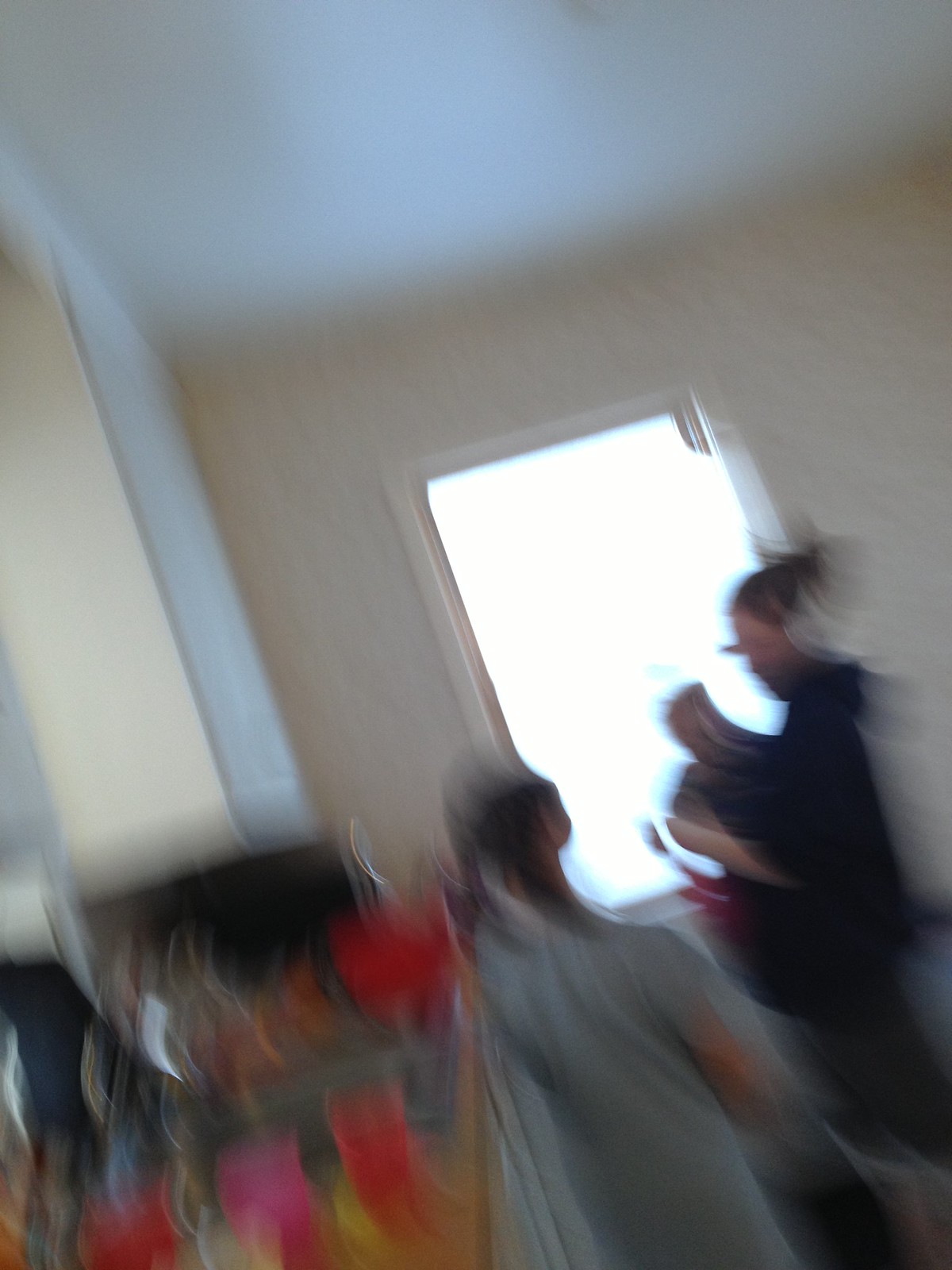A very blurry photograph captures two figures standing by a brightly lit window in a house. The image is difficult to discern due to its poor quality, but key details are visible. Both individuals appear to have dark hair; one is a child in a gray t-shirt, standing directly in front of the window. Beside the child, likely an adult woman with her hair up, is seen in a dark blue or black hoodie and gray pants. She seems to be holding something, possibly a smaller child. The room features light tan walls and a white ceiling. To the left of the figures, there is a divider or counter with an assortment of colorful cups, including red and pink. The window, which is the focal point of the image, has no curtains or blinds, allowing a significant amount of light to enter the space.